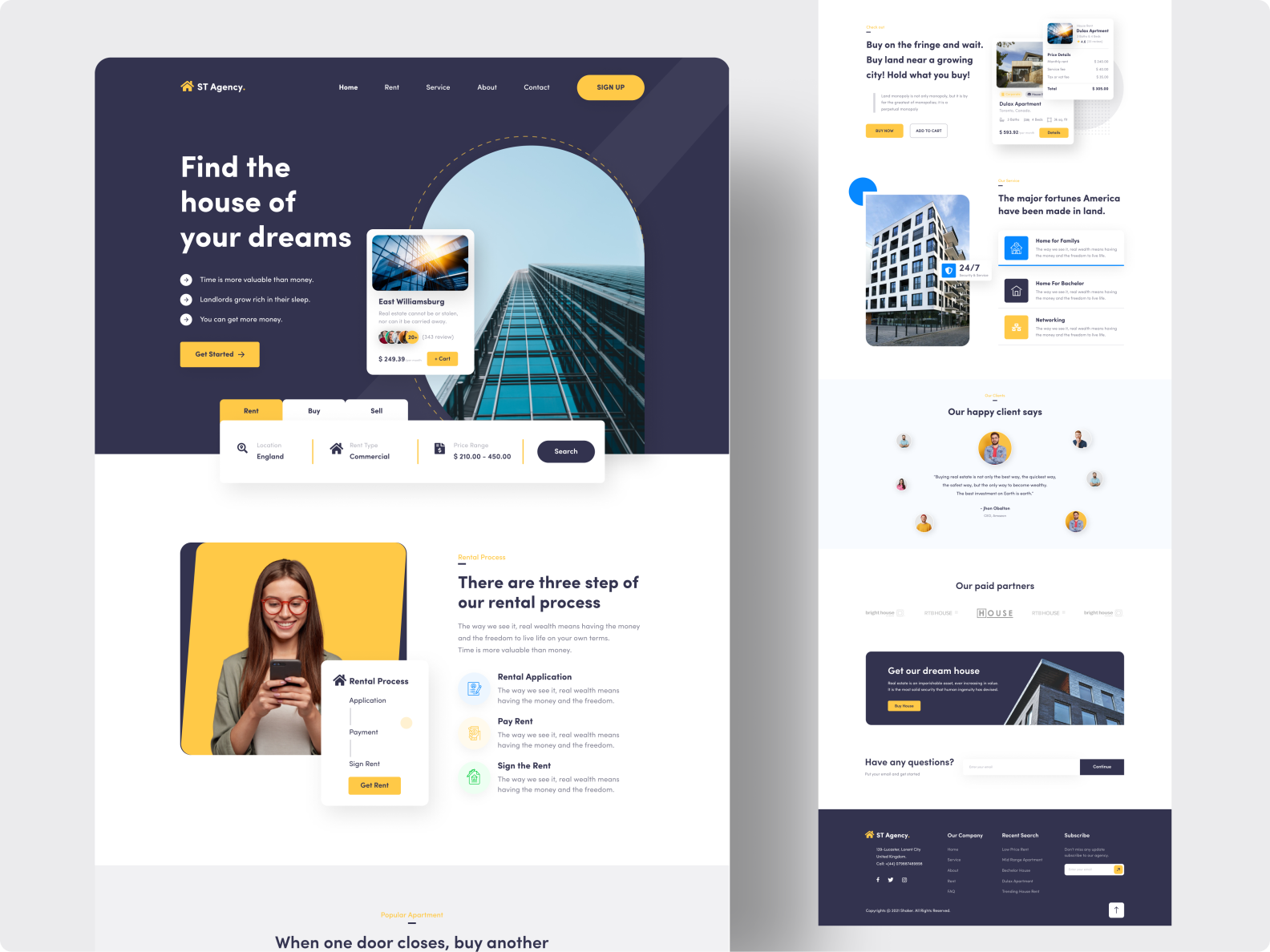**Caption:**

The image showcases the interface of an app called "ST Agency." In the top left corner, a yellow house icon is accompanied by the text "ST Agency" in white, with "ST" in capital letters. The top navigation bar features options for Home, Rent, Service, About, and Contact. On the far right, a yellow oval button labeled "Sign Up" invites users to register.

Below the navigation, a prominent headline reads "Find the house of your dreams" with three sub-options, each marked with a white circle and an arrow:

1. Time is more valuable than money.
2. Landlords grow rich in their sleep.
3. You can get more money.

A yellow button with black text and an arrow labeled "Get Started" is prominently displayed. An option for "East Williamsburg" is shown, though the text is too small to discern clearly. Users can choose between Rent, Buy, or Sell, and the default location seems to be England. The selected rent type is Commercial with a price range from $210 to $450. A black oval button with white text labeled "Search" facilitates the search process.

The lower portion of the image features a young woman with dark brown hair parted in the middle, wearing straight, shoulder-length hair. She is smiling while looking at her phone. Her red, large-framed circular glasses stand out against the yellow background.

Adjacent to her image are steps of the rental process: "Rental Process," "Application," "Payment," and "Sign Rent." A button labeled "Get Rent" is also present. Each rental process step is accompanied by the repeated phrase: "The way we see it, real wealth means having the money and the freedom to live life on your own terms. Time is more valuable than money."

At the very bottom, the text "Popular Apartment" is displayed alongside the motivational statement: "When one door closes, buy another."